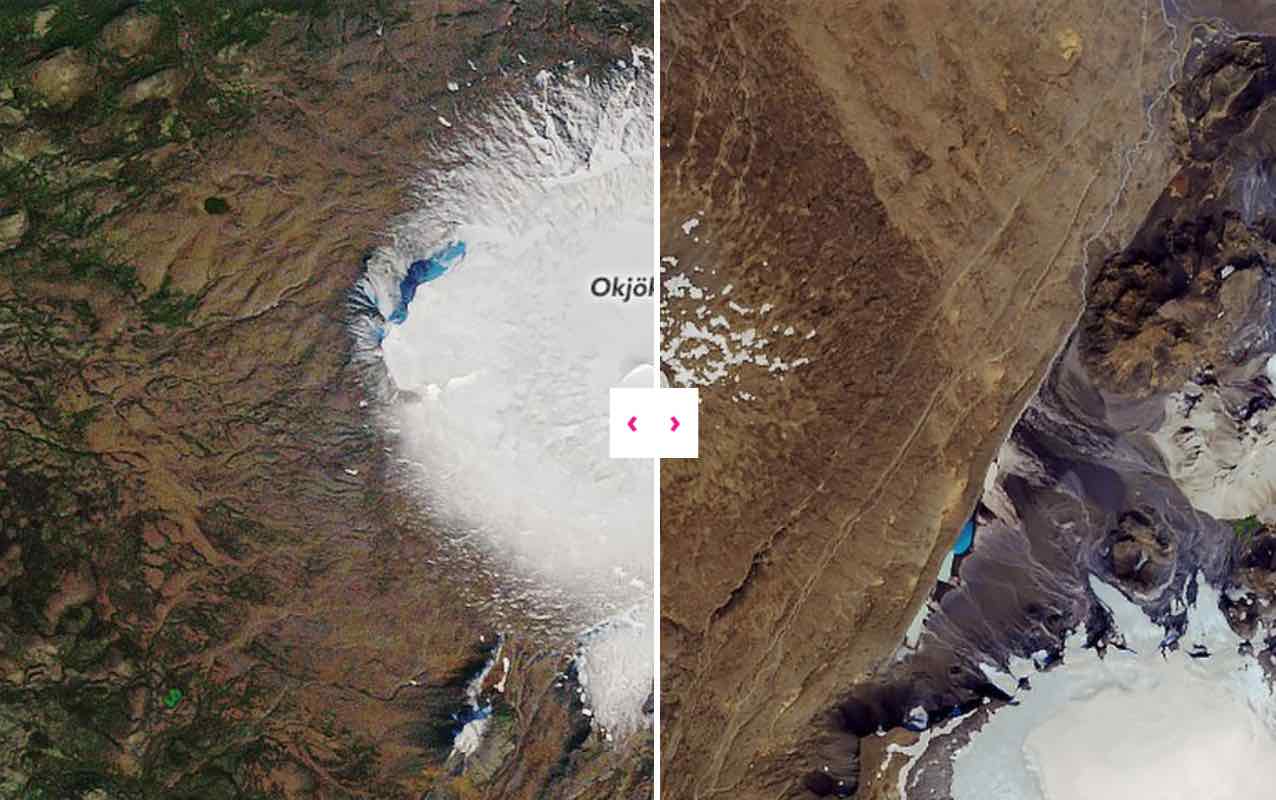The image consists of two separate overhead geographic snapshots, divided by a white line with a white box containing pink arrows indicating the possibility of swiping left or right for different views. Each side showcases distinct landscapes. The left image predominantly features green and brown terrain, with a significant icy white area to the right. This section appears mountainous with visible rivers, suggesting a high-altitude perspective. Contrastingly, the right image is more uniformly brown but also contains a noticeable white icy or rocky section in the bottom right corner. The overall presentation hints at an interactive feature, though this particular instance is a static screenshot.